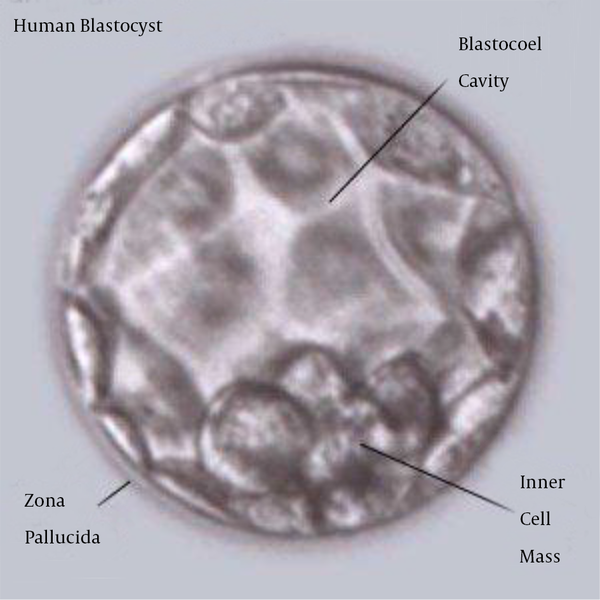The image depicts a detailed, grayscale, and slightly blurry microscopic photograph of a human blastocyst, with a gray background. The circular cell takes center stage, showcasing various organelles and structural components differentiated within its rounded shape. The edges of the cell exhibit a darker purplish-gray hue, transitioning to smoother light gray and almost whitish tones towards the center. Notable features include a cluster of mostly circular organelles and some geometrically dark patterns with white lines around them. Labeled annotations in black text identify key parts: "human blastocyst" at the top, "blastocyst cavity" pointing to a central cavity, "inner cell mass" labeling a clustered area of organelles, and "zona pellucida" marking the outermost region of the cell.